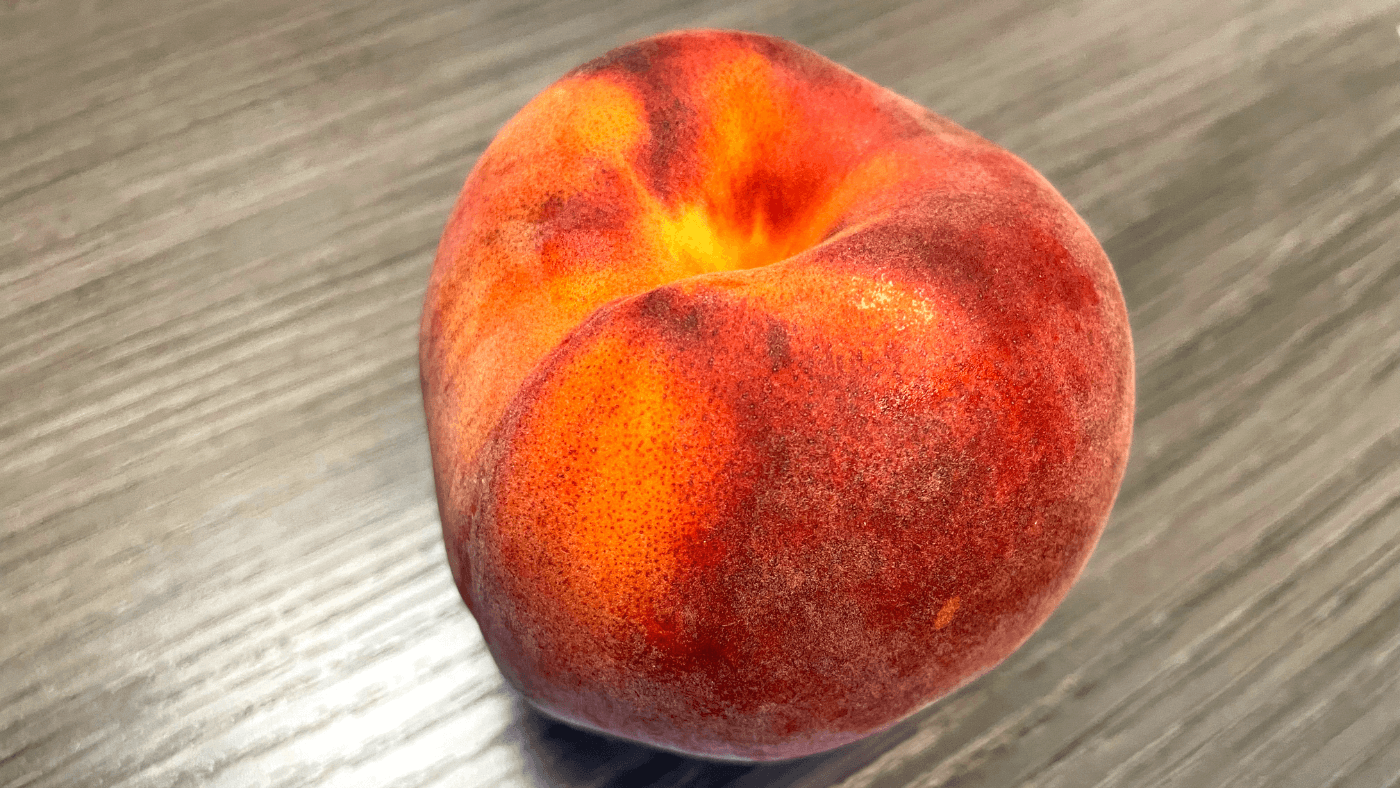This detailed image showcases a vibrant fruit, likely a nectarine due to its smooth skin, though it closely resembles a peach. Captured from above, the nectarine dominates the center of the photograph, nearly filling the frame. It displays an array of rich hues, including deep reds, oranges, and touches of bright yellow, highlighting its freshness and readiness to be eaten. The nectarine is set against a wooden tabletop surface that appears brown or gray in color. The fruit is highly detailed, and there's an almost artistic quality to the photo, with its realistic colors and textures giving the impression that it could easily be a meticulously crafted still life drawing. No text accompanies the image, and the overall presentation emphasizes the simplicity and beauty of the single nectarine resting on the table, making it an appealing subject for a future meal or snack.